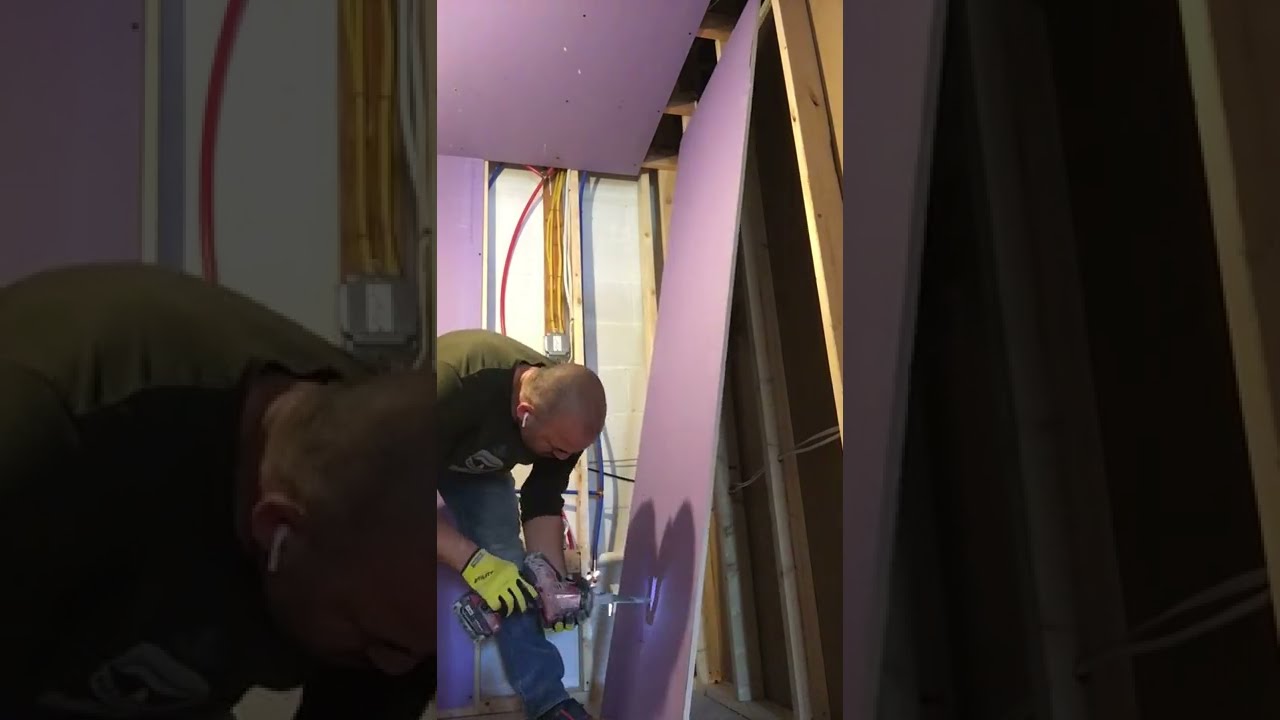In the center panel of this triptych photograph, a middle-aged bald man with white earplugs is bent over at a 45-degree angle, wearing an olive green t-shirt with sleeves pushed up and blue jeans. He is holding a jigsaw in his yellow-gloved right hand, operating it on a large light purple board in front of him. The room's walls are unfinished, revealing wood framing, exposed cement blocks, and various wires running top to bottom. The lavender-purple ceiling matches the board on which the man is working, indicating ongoing renovations. The left inset of the photograph shows a close-up of the man's head, while the right inset displays a detailed view of the board, with both insets presented in a darker, gray tone compared to the brightly colored center panel.